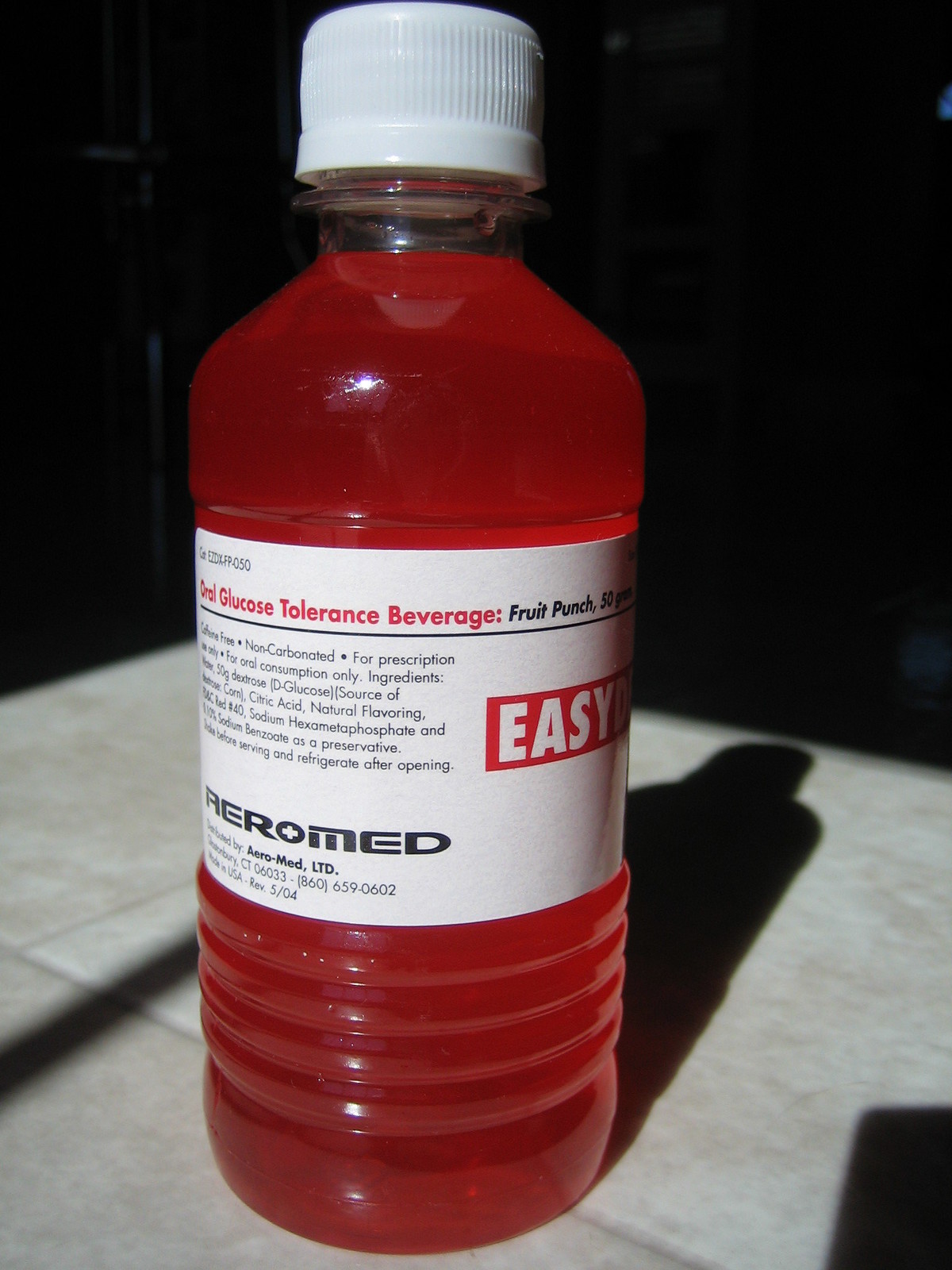This vertically rectangular image is well-lit from the upper left, casting a pronounced shadow behind its subject—a medium-height, clear plastic bottle with a white lid. The bottle is filled with a vibrant red liquid, presumably a beverage. Wrapped around the center of the bottle is a white label, partially capturing text from both its front and back. The label's red lettering prominently reads, "Oral Glucose Tolerance Beverage," while beneath, "Fruit Punch" is inscribed in black. Towards the bottom of the label, additional black text appears to spell out, "Pure Med." The composition and sharpness of the shadow accentuate the bottle's presence within the frame.